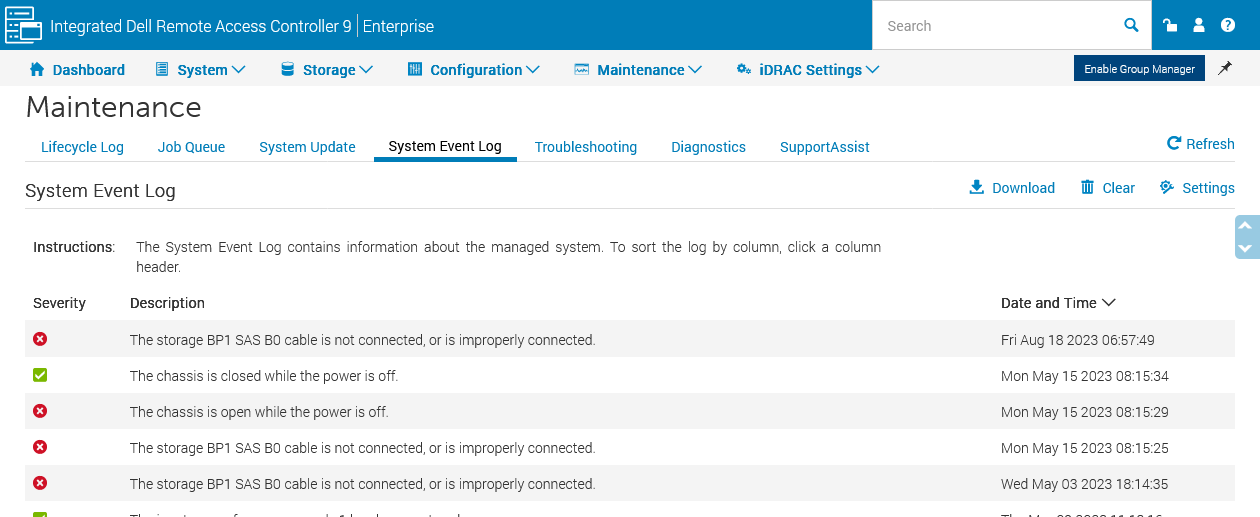The image displays a webpage featuring the Integrated Dell Remote Access Controller 9 Enterprise interface. At the top of the page, a thin blue bar contains a maintenance menu, with a search bar situated just below. Directly beneath the search bar, a row of primary menu options is visible: Dashboard, System, Storage, Configuration, Maintenance, and IDRAC Settings.

The Maintenance section is prominently highlighted, revealing a series of tabs associated with it: Life Cycle Log, Job Queues, System Updates, System Event Log, Troubleshooting, Diagnostics, and Support Assist. The focus is on the System Event Log tab, which details various system events.

Each entry in the System Event Log is organized into columns, displaying the event's severity (with icons indicating either a red circle for severe issues or a green box with a checkmark for issues that have been resolved or are non-critical), a brief description of the event, and the specific date and time the event occurred.